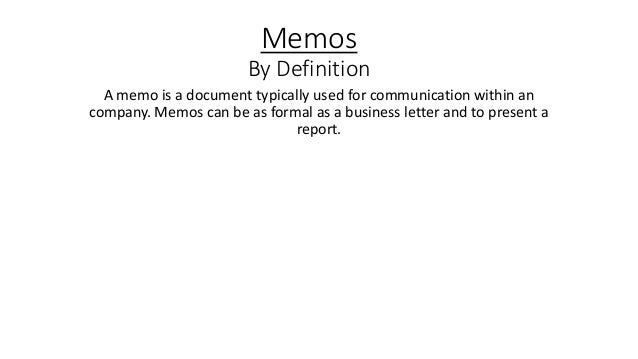The image features a slide from a PowerPoint presentation with a blank white background. At the top, centered in bold black text, is the word "Memos," which is both capitalized and underlined by a thin black horizontal line. Directly beneath this, in black lettering, is the heading "By Definition," with both the B and D capitalized. The accompanying text reads, "A memo is a document typically used for communication within a company. Memos can be as formal as a business letter and to present a report." The text is presented in a thin, easy-to-read font, giving a clear and straightforward definition of what memos are. The slide appears to be designed to convey the official textbook-like definition of a memo.